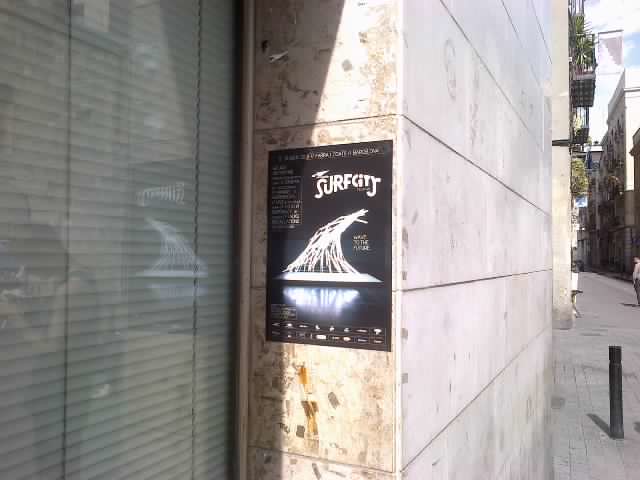The image depicts the side of an exterior wall of a building on a sunny day. The wall, mostly white with a hint of yellow where the sun strikes it, runs adjacent to a gray sidewalk. To the right, the smoother expanse of the wall shows a bit of shadow. On the side of the wall, there's an indentation housing a window with visible lines and reflections, including a blurry figure that appears to be a lady working at a countertop. To the left of the image, we see an alleyway characterized by a shadowed, skinny, yet lit passage which appears to be blocked off by a black post. In the center of the wall, there is a prominently displayed black poster. The top of this poster features the words "Surf City" in bold white letters. Below, the rest of the text, mostly illegible and in another language, accompanies a striking image resembling a leaning teepee or wave curving to the right. The teepee-like object reflects off the surface beneath it, suggesting it’s mirrored on something smooth, dark, and glossy like black ice.